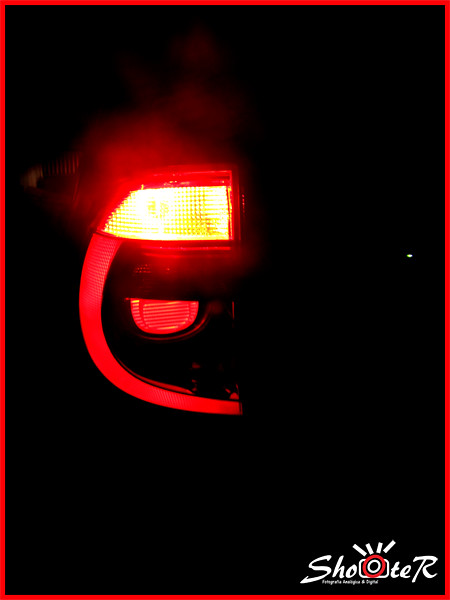The image features a black background with a single illuminated left taillight of an unidentified vehicle, indicating that it is nighttime. The taillight, glowing bright red, creates a red mist and is framed by a striking red border. Below the taillight, a red streak curves downward, creating a facial-like effect. In the lower right corner, the branding "Shooter" appears in white font, with a red ring around the second "O" and a small white rectangle with four lines emerging from its top. Fine print in white font is visible beneath the branding, likely indicating the company responsible for the photograph.